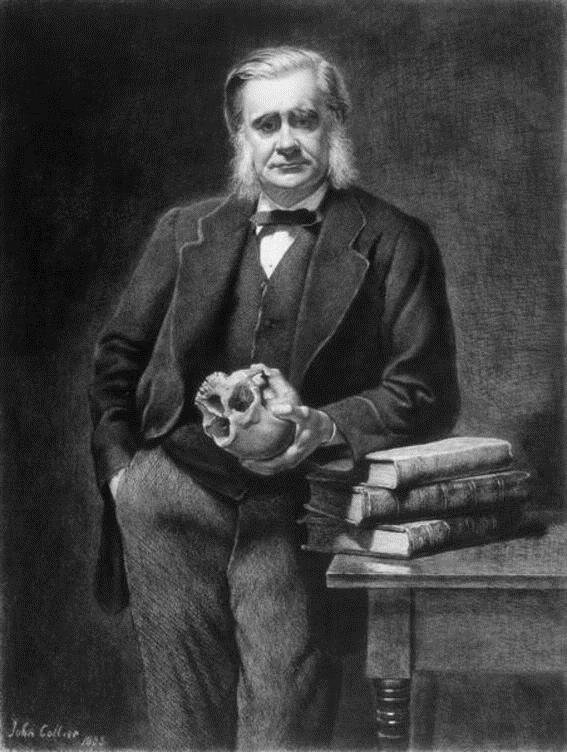This is a detailed black-and-white artwork by John Collier, presumably created around the late 19th or early 20th century, depicting an older white man with distinct features and attire. The man's hair, a mix of gray and white, is neatly parted to one side and extends down to his shoulders, with prominent, fluffy sideburns framing his face. He has no facial hair and sports bushy eyebrows, contributing to his mature and somber expression as he gazes straight ahead.

Dressed in classic formal attire, the man wears a black suit jacket, a black vest, a white dress shirt, gray slacks, and a black bowtie. His right hand is tucked into his right pocket, while his left elbow rests on a stack of three books placed on an old-fashioned wooden table to his right. In his left hand, he holds a human skull, grasping it upside down at the top, evoking both a scholarly and contemplative air.

The background of the image is a stark, blackish-gray, devoid of any other objects or figures, focusing all attention on the man and his contemplative pose. In the bottom left-hand corner, there is a signature, "John Collier," though the accompanying date is difficult to decipher, possibly reading 1935, 1905, or 1883.